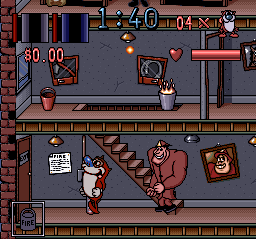In this cartoon-style image, which seems to be a screenshot from a video game, we see a two-level interior setting. The environment is rendered in slate gray tones, covering the walls of both the top and bottom floors. Central to the lower floor is a brown staircase that connects the two levels. 

On this lower level, two distinct characters are prominently featured. To the left, we have an anthropomorphic cat standing upright. The cat's face and stomach are predominantly white, while its back and legs display a striking orange hue. Positioned next to the staircase is a cartoonish man with an exaggeratedly large and muscular torso, and an oblong-shaped head, further adding to the whimsical atmosphere of the scene.